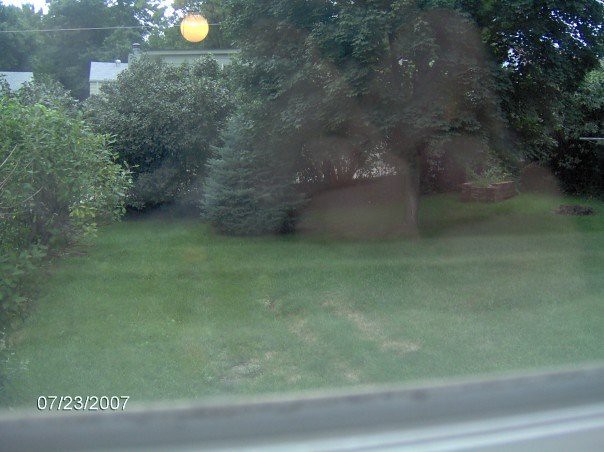A color photograph taken from the edge of a road through the windshield of a vehicle, evidenced by the faint reflections on the glass. The photograph is dated "7-23-2007" in white text at the bottom left corner. The lower part of the image features a blurry road marked by thin white lines. Beyond the road, there is a grassy lawn area with a backdrop of shrubs, more brightly illuminated on the left side. A white building partially obscured by the shrubs is visible on the left, with a prominent, round, yellow light above it. This light appears to be illuminating the surrounding foliage. To the right, raised flower beds create an alcove-like arrangement, though some details may be distorted by reflections from the vehicle.